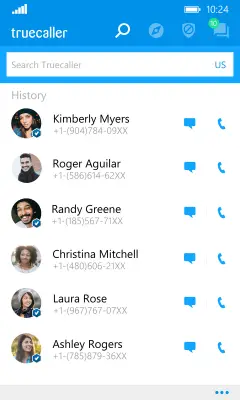The image is a screenshot of the Truecaller app interface. At the top, there is a light blue header that features the signal strength icon on the left and the battery icon along with the time displayed as 20:24 on the right. Below the header bar, the Truecaller search icon is visible. The main section of the screenshot lists several contacts including Kimberly Myers with her phone number prominently displayed along with icons for messaging and calling options. Additional contacts listed on the Truecaller history page include Roger Akila, Randy Green, Christina Michelle, Laura Rose, and Ashley Rogers, each accompanied by their respective phone numbers.